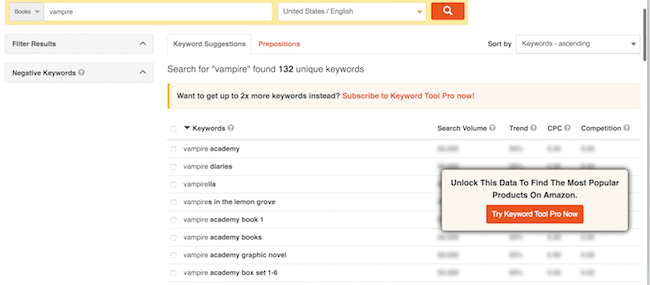The image depicts a webpage interface dedicated to book searching and keyword analysis. The page, primarily white with subtle orange highlights including the search magnifying glass button, appears to belong to a keyword research tool. The user has selected the "Books" category and typed "vampire" into the search bar located in the top left corner. They have also set the regional filter to "U.S./English."

The left panel features options to filter results and negative keywords, both of which are currently collapsed. While the term "negative keywords" is not explicitly explained, it is likely intended to exclude results containing specified words.

The search results indicate that the keyword "vampire" yielded 132 unique keywords. Prominent book titles in the results include "Vampire Academy," "The Vampire Diaries," "Vampirella," "Vampire in the Lemon Grove," and "Vampire Academy Book 1."

To the right of the search results, a table displays metrics such as search volume, trend, CPC (cost per click), and competition. However, detailed data for these metrics are locked behind a prompt encouraging users to try "Keyword Tool Pro" to unlock the most popular product insights on Amazon.